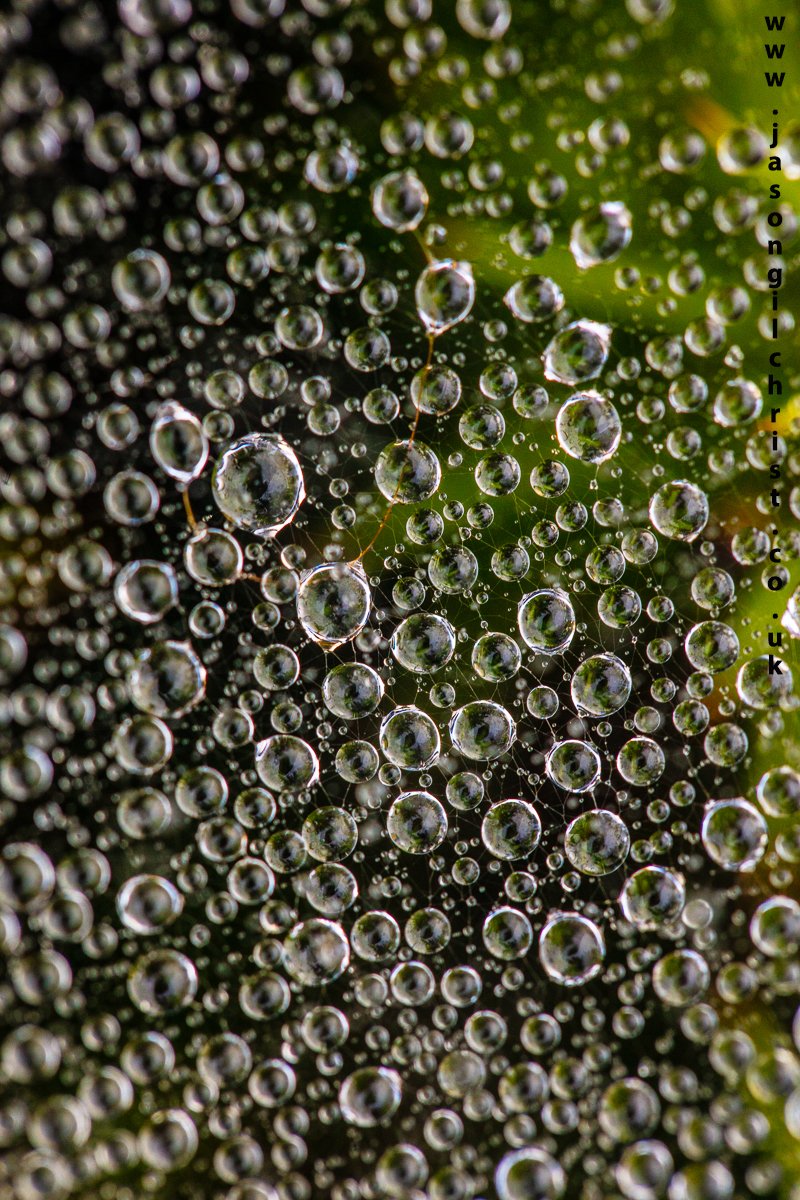The image showcases an intricate cobweb adorned with numerous water droplets of varied sizes, creating a visually striking pattern against a predominantly dark background with subtle hues of green and yellow. The droplets, resembling transparent bubbles, are clustered densely, with each one reflecting light and a spectrum of colors, particularly green. The web itself is accentuated by delicate, thin white lines that weave through and between the droplets, highlighting the moisture. The outer edges of the droplets are notably reflective, capturing light from the right side. The image is marked by a text at the top right corner, reading "jasongilchrist.com.uk," indicating the photographer's credit.